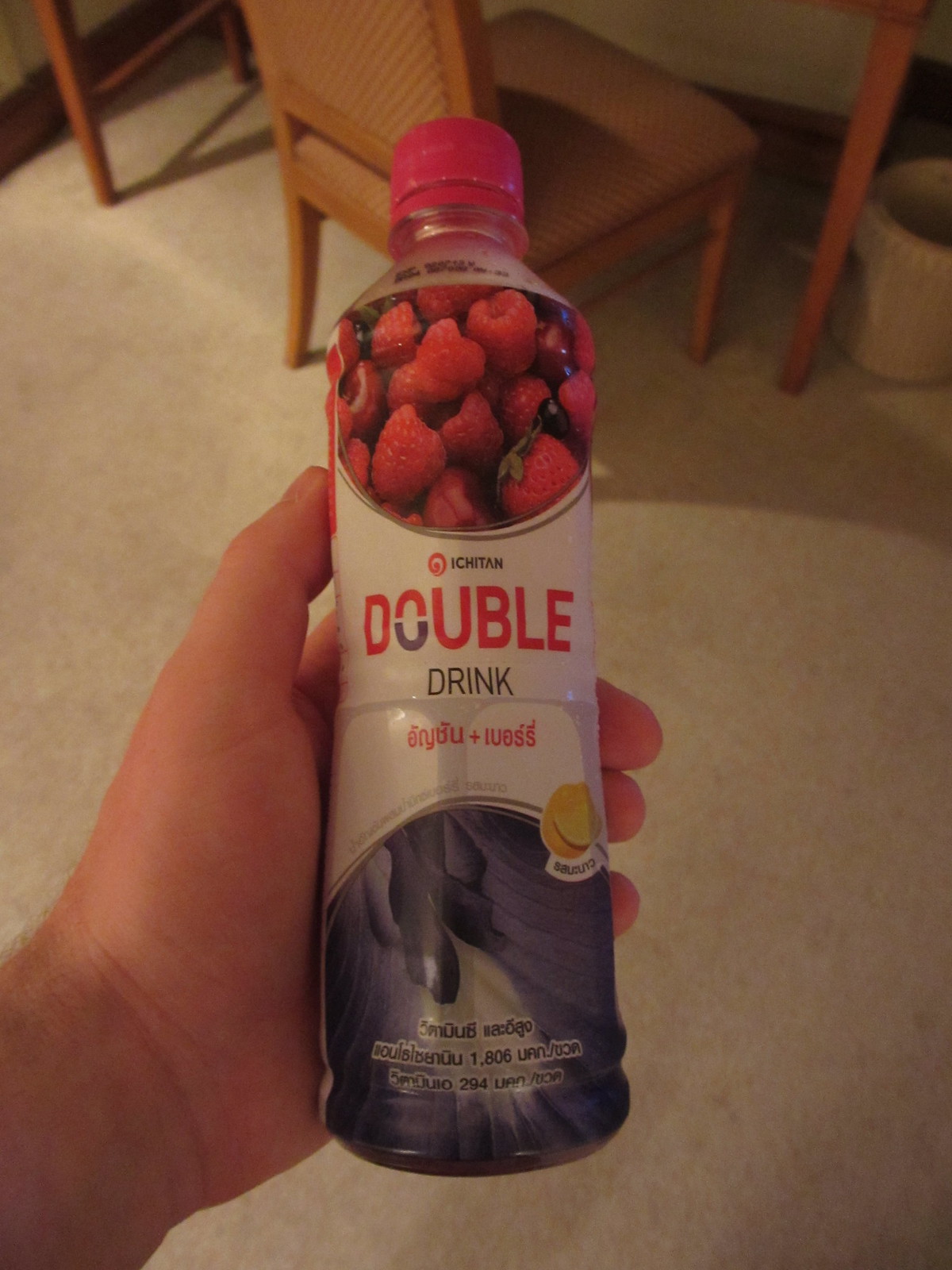The photo, taken indoors, features a setting with a white tiled floor. In the upper part of the image, a wooden leg of a table is visible, next to an empty paint canister. There's a wooden chair positioned at the table, showcasing a woven design on its back. On the left side of the photo, a person's fair-complexioned, hairy arm can be seen, holding a plastic bottle with a red top. The bottle prominently displays raspberries and bears the label "Ishitan Double Drink." Beneath the main text, there is additional writing in what appears to be Thai or Cambodian, located inside a gray or purple area.